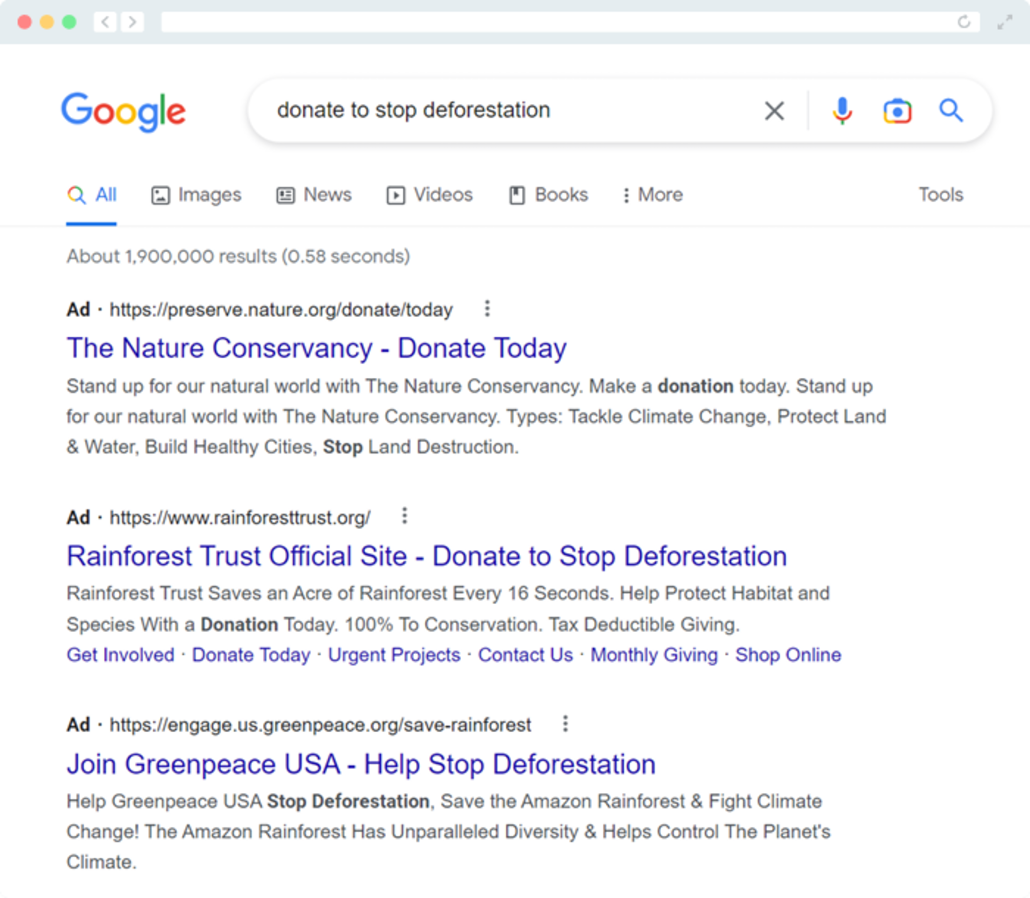### Websites

**Google Search Page: Donations to Stop Deforestation**

The image features a Google search results page. Prominently displayed at the top left corner is the iconic Google logo. The search bar contains the query "donate to stop deforestation." Adjacent to the search bar are several utility icons, including an 'X' to clear the query, a microphone for voice-to-text input, a camera icon for image search, and the ubiquitous magnifying glass to initiate the search.

Below the search bar is a series of navigational tabs: "All," "Images," "News," "Videos," "Books," "More," and "Tools." These allow users to refine their search results based on content type.

The first set of search results primarily consists of advertisements related to donating to stop deforestation:
- **Nature Conservancy**: The top ad urges viewers to "Donate today, stand up for our natural world with the Nature Conservancy. Make a donation today."
- **Rainforest Trust**: The next ad promotes the "Rainforest Trust official site" and highlights that they "save an acre of rainforest every 16 seconds. Help protect habitat and species with a donation today."
- **Greenpeace USA**: The final ad in the sequence calls for action to "Help stop deforestation. Save the Amazon rainforest and fight climate change by joining Greenpeace USA."

These ads collectively emphasize the urgency and importance of contributing to efforts aimed at halting deforestation and protecting our natural environment.